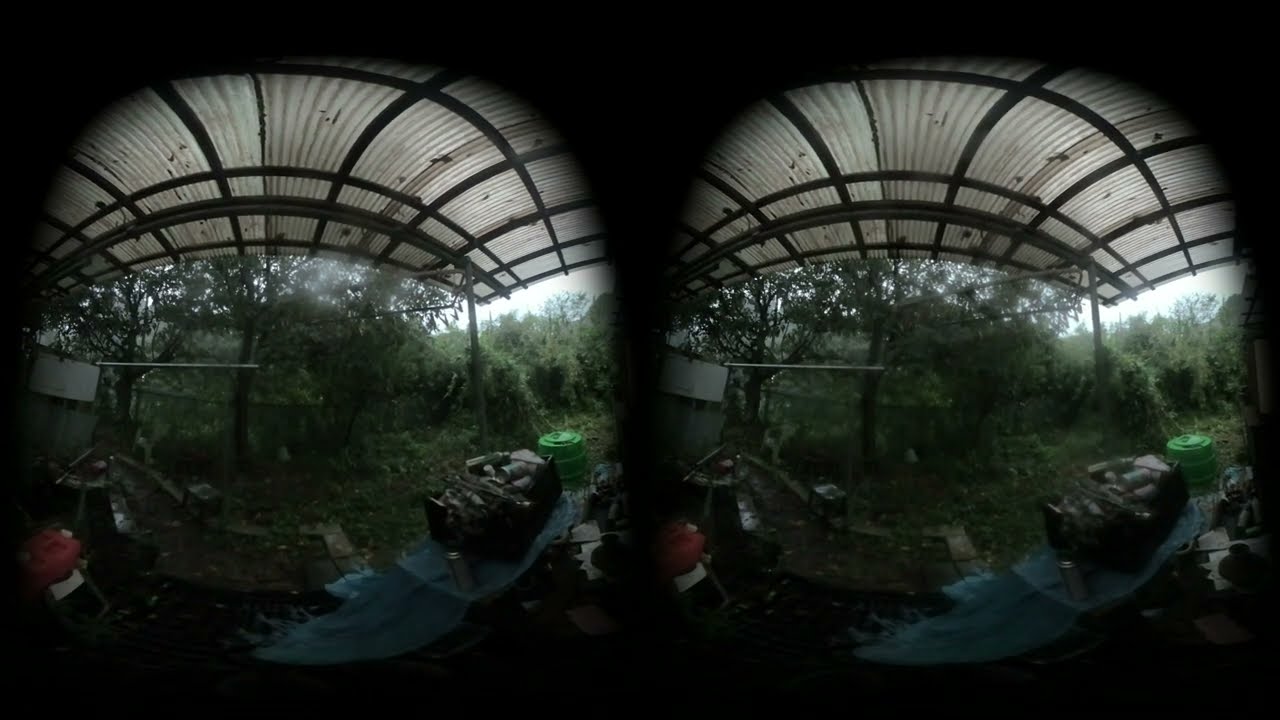The image depicts a symmetrical scene, split equally down the middle as if viewed through a vintage stereo viewfinder or binoculars, characterized by dark borders framing two identical circular visuals. Both sides show a dilapidated setting with a curved, corrugated plastic or tin roof supported by metal rafters. This structure, resembling a carport with no visible walls or doors, shelters various debris and items. Among these, a red gas can sits on the extreme left corner, noticeable through its lighter-colored cap, while a green barrel is positioned towards the right middle. Scattered rocks, bricks, and dirt cover the ground beneath this makeshift canopy, along with a disordered mix of containers, bins, and possibly a tarp or drop cloth at the bottom. Surrounding the area is an untamed backdrop of green trees and shrubs, suggesting this might be an unkempt backyard setting. The sky is bright, yet its color and the presence of the sun are indiscernible.